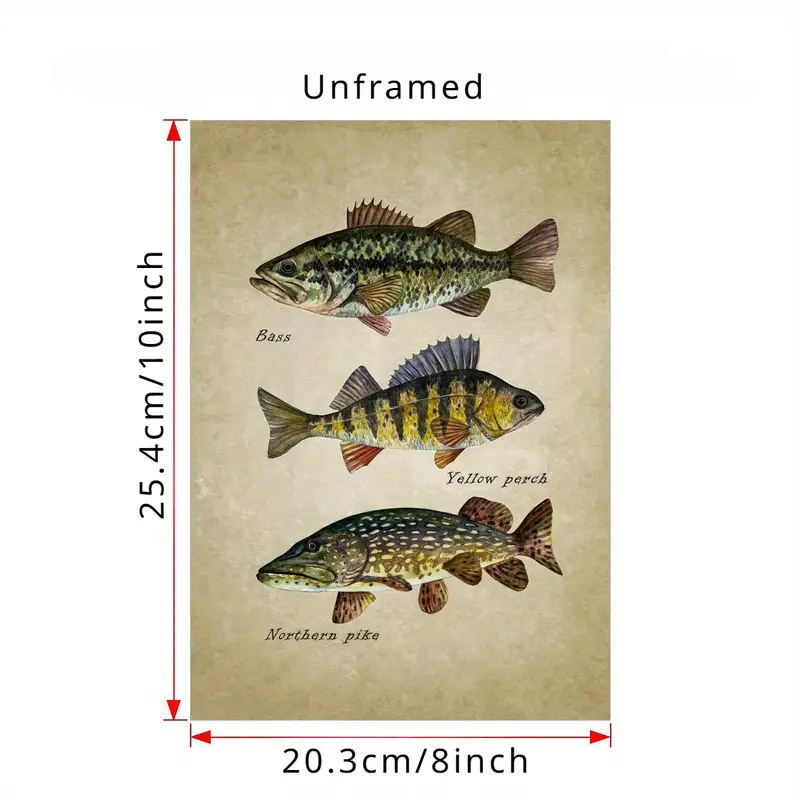This is an unframed poster that features three fish illustrated side-by-side against a pale, antique-like background, reminiscent of an old textbook or vintage book illustration. The overall dimensions of the poster are marked with red arrows: 25.4 centimeters (10 inches) in height and 20.3 centimeters (8 inches) in width. At the top of the poster, the word "unframed" is clearly labeled in black lettering.

The fish are depicted with meticulous detail, showcasing their distinctive colors and patterns. 

- **Top Fish: Bass**  
  The bass is facing to the left. Its body is primarily green with black stripes or spots and has a white underbelly. The mouth of the fish is slightly open, and the fins, including a spiky dorsal fin and a fanned tail, are a grayish-brown color, with some depictions mentioning they have brown and black markings. This fish is labeled "bass" underneath its mouth in black text.

- **Middle Fish: Yellow Perch**  
  The yellow perch is oriented to the right. Its body is a bright yellow with green or black tiger-like stripes running vertically down its side. The fins are vividly colored, with purplish or reddish fins near the gills and a yellow and green tail. It has a light blue patch around its eyes and a spiky blue dorsal fin, with a flatter fin beneath it. The labeled text "yellow perch" is found below this fish.

- **Bottom Fish: Northern Pike**  
  The northern pike has its head facing to the left and displays a dark green body adorned with numerous white speckles and some short stripes. Its underbelly and underside of the mouth are white. This fish features a long, flat mouth and a relatively flat face, with several fins displayed in varying shades of brown, gray, and even maroon, all marked with black specks. This includes a significant tail fin that is fanned out. Underneath this fish, the label reads "northern pike."

Each fish is drawn with a side view and colored with distinct patterns that highlight their species, from the green hues of the bass to the vibrant yellow and green of the yellow perch, to the speckled patterns on the northern pike.